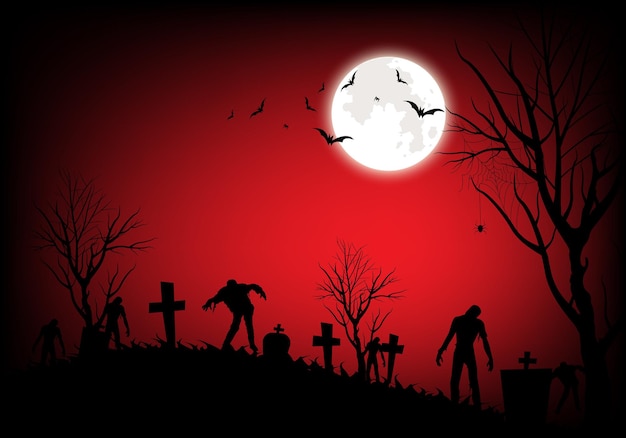This eerie nighttime scene is rendered in a cartoon style with a haunting red gradient background that deepens to near-black at the edges and brightens to a vibrant red towards the center. Dominating the upper center of the image is a large, glowing full moon, adorned with subtle gradients from bright white to a slightly tan hue, emulating the natural look of craters. Black silhouettes of at least ten bats can be seen flying around and in front of the moon.

In the cemetery set on a dark, moonlit hill covering the bottom half of the image, numerous cross-shaped tombstones stand solemnly amidst sparse, leafless trees on both sides. To the right, one barren tree even hosts a black spider descending from a branch. Silhouetted zombies and monsters are scattered among the tombstones, adding to the creepy atmosphere. The foreground, drawn in stark black, enhances the ghastly feel of the scene, with ominous shadows casting across the cemetery under the eerie moonlight.